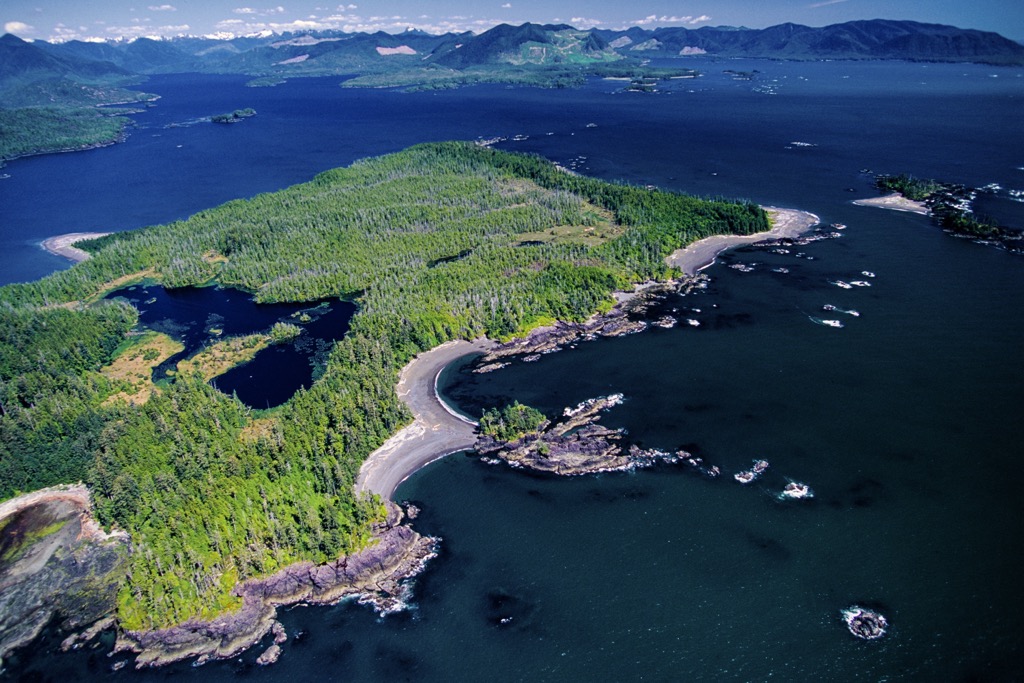This aerial photograph captures a stunning coastal landscape that may resemble regions like Vancouver Island, Alaska, or even the Galapagos Islands. The image showcases a rugged and diverse geographical area marked by towering, mountainous terrain in the background, some of which appear to have volcanic origins due to their pointed peaks. The mountains trail off to the right, merging into steep cliffs adorned with dense greenery. 

Central to the image is a unique land formation with a roughly rectangular shape, though irregular in its outline. This area is mostly covered with lush, dark green conifer trees and pathways that look like dirt roads winding through the terrain. The perimeter is a mix of rocky shores and patches of grayish sand that meet the deep, dark blue ocean waters.

The coastline is dramatically rocky in places, with the sea crashing against large boulders, creating visible white surf marks. In the top center, flat areas transition into more elevated, vegetated regions. There's a distinct inlet on the left side, suggesting the presence of smaller islands within the expansive water body, with the ocean dotted by scattered rock formations.

Above the mountains, a light cloud cover adds to the serene atmosphere. Prominently, a small pond is nestled within the central green area of the land formation, completing the picturesque and richly textured scene.